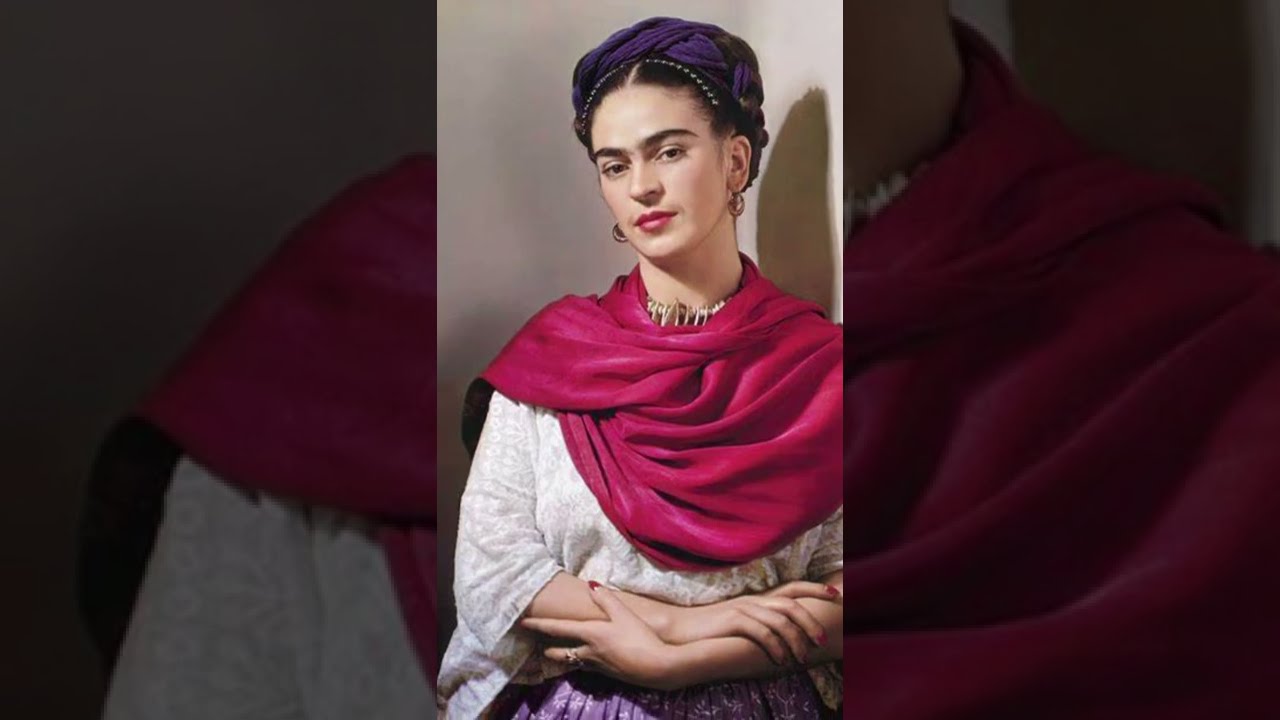This old-school portrait features a woman, possibly in her 20s, with striking similarity to Frida Kahlo. She has dark hair and prominent, unaltered eyebrows, highlighted by the red lipstick she wears. Her head is slightly tilted to the left, adorned with a dark purple turban or scarf, complete with beads along the bottom. Dangling earrings are visible from either ear. Her attire includes a vibrant scarlet shawl draped over her shoulders, beneath which she dons a white peasant blouse with sleeves extending past her elbows. She also wears a distinctive necklace with metal bars. Her arms are clasped in front of her, each hand holding the opposite forearm. The purple pleated skirt she wears peeks out at the bottom of the image. The background features a faint shadow of her head on a wall, contrasting against a slightly darker gray area. The composition includes a blurred border to the left and right, enhancing the central focus on the woman and her detailed, colorful attire.